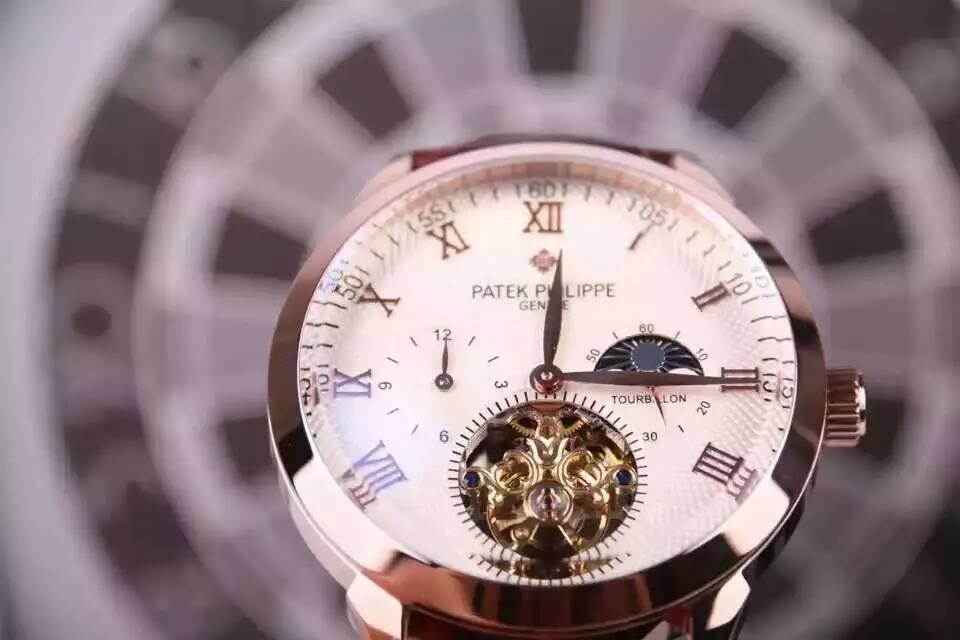This image features a sophisticated and intricate Patek Philippe watch. The backdrop of the photograph is a dartboard with a brown and white design, adding an interesting contrast to the timepiece. The watch itself showcases a bronze-colored case, adding to its luxurious appearance. The face of the watch includes Roman numerals in the same bronze hue for the hour markers, while the minute markers are in black. The brand name "Patek Philippe" is prominently displayed on the dial, partially obscured by the hour hand. The watch currently reads approximately 12:15.